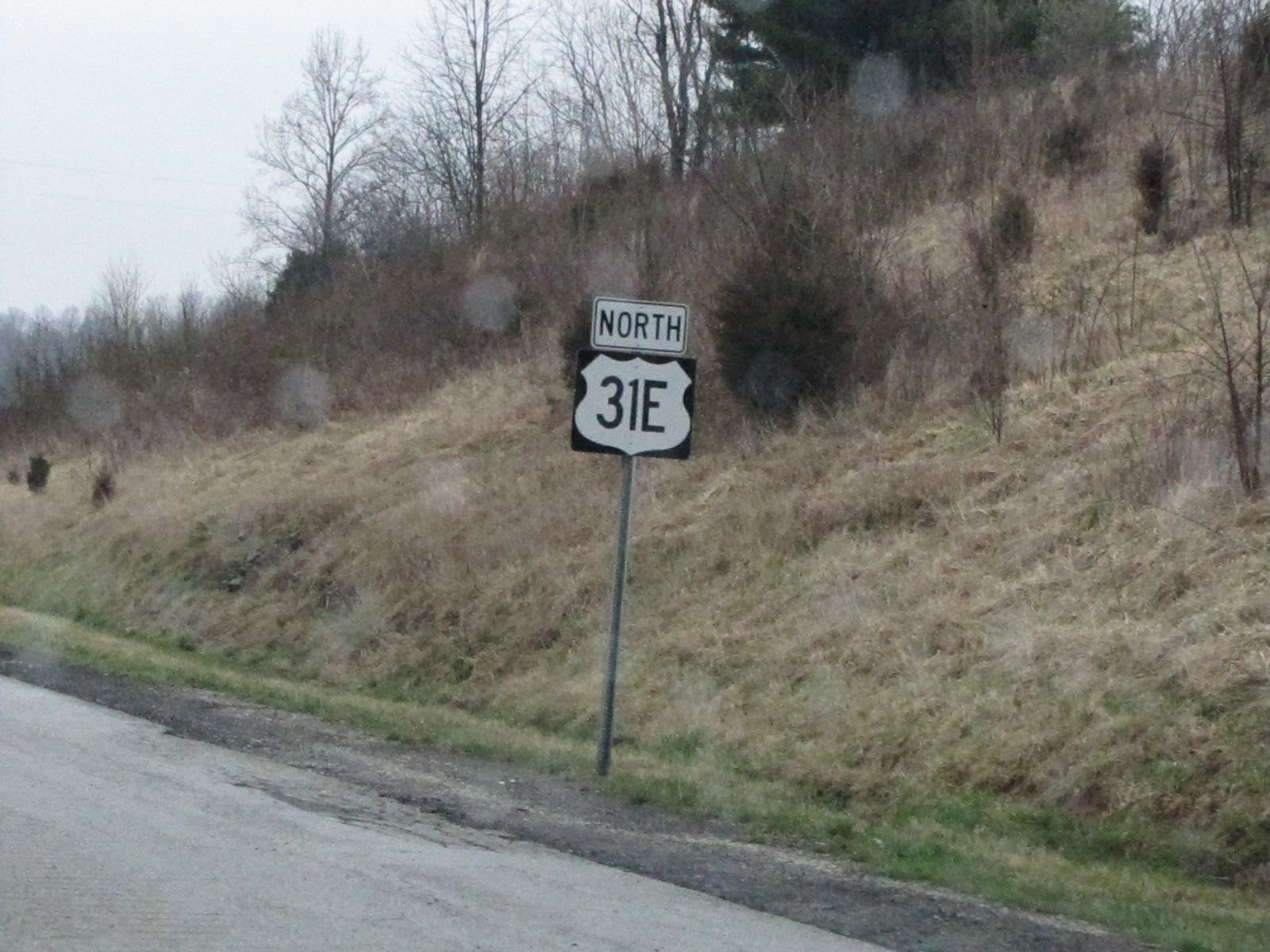In the foreground of the image, there's a prominent black and white street sign on a single silver pole, positioned at the side of a seemingly less-traveled road. The sign displays "North 31E" in bold black letters, with "North" on a smaller rectangular sign above the larger "31E" sign. The road itself appears worn, composed of gravel and gray asphalt bordered by a black strip which could be dirt or concrete. Just beyond the edge of the road, dried and yellowed grass extends upwards into a hill, interspersed with patches of light green grass and a few dark green bushes.

The backdrop is dominated by a consistent winter scene, characterized by leafless trees, with one large evergreen or pine tree standing prominently on the hill. Most of the background is filled with smaller, younger trees scattered around the hillside. The sky overhead is a bright, light gray, indicative of a cloudy and overcast day. The overall atmosphere suggests a cold, possibly wintery day in a small town area.